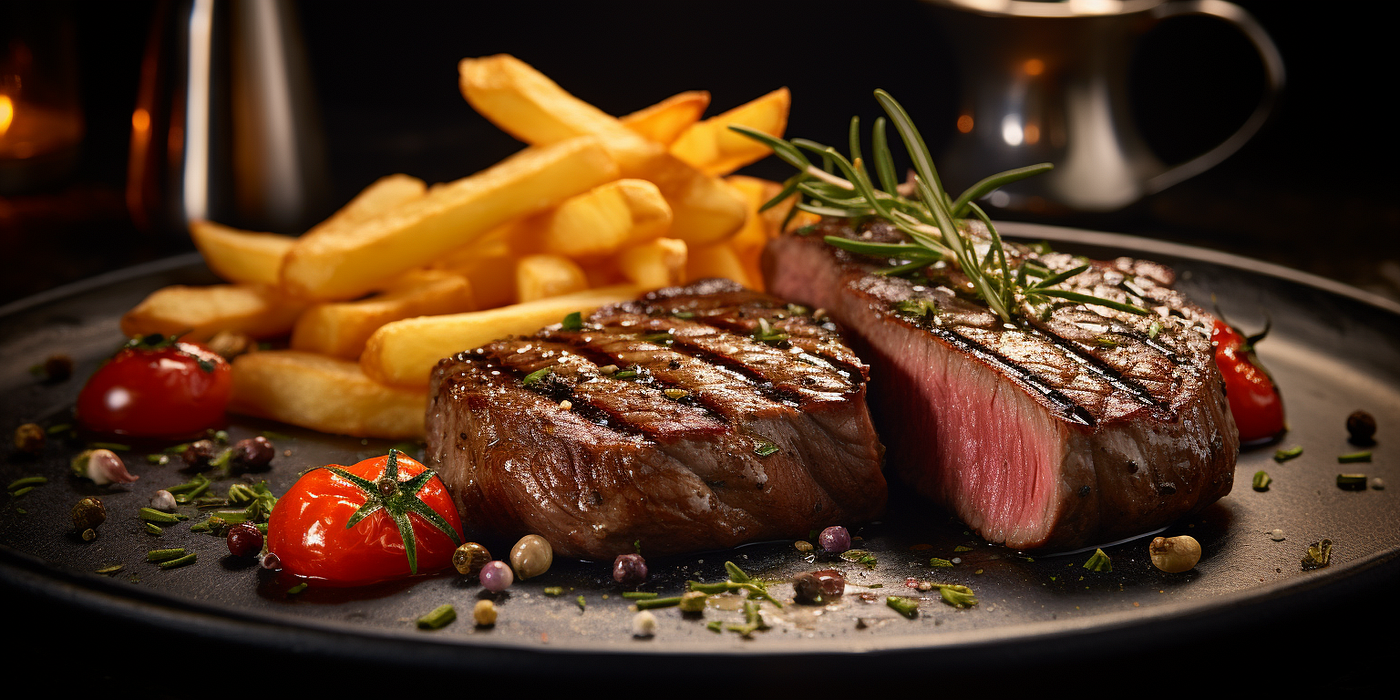This is a highly detailed professional photograph of a plated dish, likely taken at a restaurant. The focal point is a seared New York sirloin steak, presented on a round, metallic black plate. The steak, cut into two non-matching, perpendicular pieces, is cooked to a medium-rare doneness, featuring a red and pink center with a hint of gray near the edges. Prominent grill marks and a dark brown sear enhance its visual appeal. The steak is garnished with a scattering of fresh rosemary sprigs and small thyme leaves. Surrounding the steak are three half-cut tomatoes, showcasing green stems, along with several juniper berries that add pops of purple and gray color. Positioned behind the steak are thick, golden yellow steak fries. The entire setup rests on a glossy black table, with a blurred background featuring a shiny metal cup with a handle and another indistinct metal pitcher, contributing to the overall restaurant ambiance.